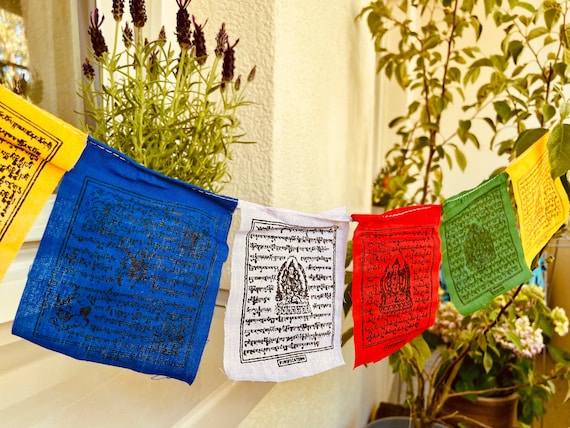The image showcases a series of multi-colored banners hanging on a rope that droops slightly in the middle, depicting their weight. The sequence of the banners from left to right is yellow, blue, white, red, green, and yellow again. Each banner features a central illustration and text that resembles Arabic script. In the background, there is a light beige-colored wall. To the left is a window partially visible, along with a building. Various plants with bright green leaves are placed in flower pots. The plant on the far left has black buds, while another, which resembles a small tree, has clusters of purple flowers, adding vibrant details to the scene.